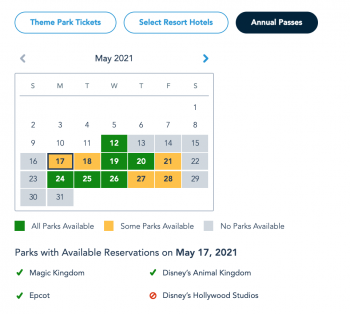The image showcases a user interface for selecting different ticket options for a theme park. At the top of the screen, there are clickable categories: "Theme Park Tickets," "Select Resort Hotels," and "Annual Passes," with the "Annual Passes" option selected, indicated by a filled bubble, while the other options remain in blue and white.

Below these options, a calendar for May 2021 is displayed, allowing navigation to future months but starting specifically at May 12th. The calendar uses a color-coded system to indicate park availability: green signifies that all parks are available, yellow denotes that only some parks are available, and gray indicates no park availability.

The detailed availability for May is as follows:
- Green (all parks available): May 12th, 19th, 20th, 24th, 25th, and 26th.
- Yellow (some parks available): May 17th, 18th, 21st, 27th, and 28th.
- Gray (no parks available): May 13th-16th, 22nd-23rd, and 29th-31st.

This interface helps visitors to plan their visits accordingly, specifically for Magic Kingdom, Epcot, and Disney’s Animal Kingdom, excluding Disney’s Hollywood Studios.